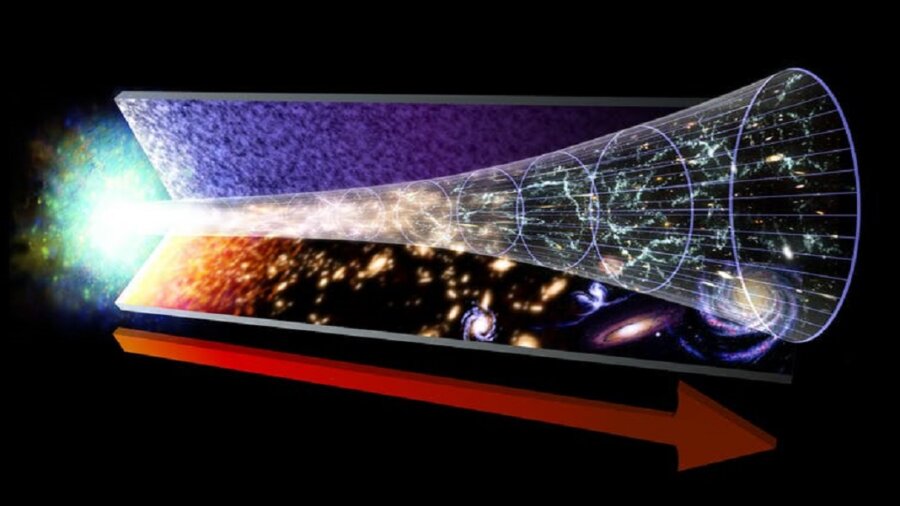The image is an illustration, possibly from a scientific context, depicting a motion or change in direction related to light or astronomical phenomena. The central figure is a transparent, trumpet-shaped or tuba-like cone that starts narrow on the left and widens towards the right. Inside the cone, horizontal white lines segment the cone into light purple ovals that gradually increase in size as they progress from left to right. These ovals are suggestive of light expanding or a wave pattern.

The background of the cone is black, speckled with star-like points, enhancing the illustration's astronomical theme. Below the cone, there is a red arrow, pointing rightward, which spans from the left to the right of the image, indicating direction or motion. Additionally, below this arrow, the imagery includes representations of celestial bodies, starting with what appears to be the sun on the left and possibly extending to different planets on the right. Above the trumpet-shaped cone, a light and dark blue surface resembles a textured wall, and to the far left, there is a cluster of very bright lights, possibly stars. The left tip of the cone disintegrates into a burst of light that transitions into teal and turquoise colors, adding to the sense of expanding light or energy.